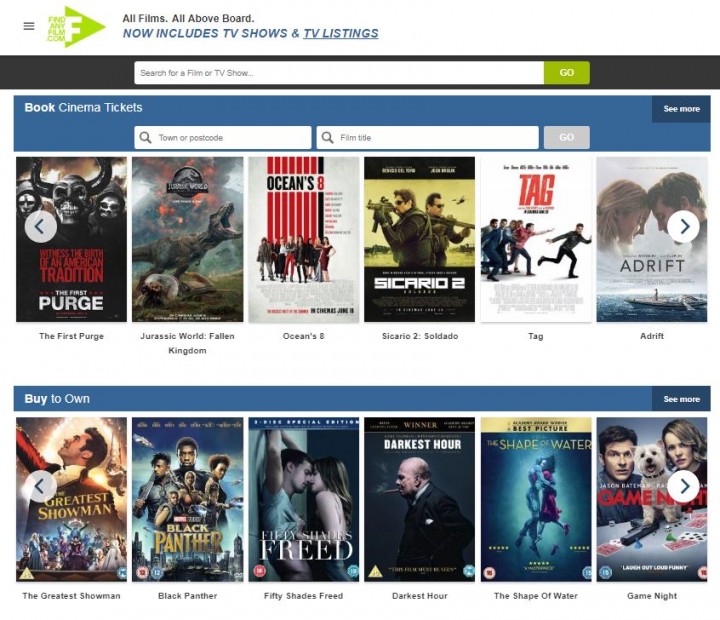Screenshot of the "FindAnyFilm.com" web page is displayed, showcasing its logo and name prominently at the top left corner, above a search bar. On the same row as the logo, there is a tagline that reads: "All films, all above board. Now includes TV shows and TV listings." Directly below this tagline is a search bar with a black background and a green "Go" button.

The web page is divided into two main sections:

1. **Book Cinema Tickets**: 
   - This section includes two search bars: one for entering a town or postcode, and another for entering a film title, with a grayed-out "Go" button to the right.
   - Under these search bars is a horizontal row of movie posters. The films featured are:
     - The Purge
     - Jurassic Park: Fallen Kingdom
     - Ocean's 8
     - Sicario 2: Soldado
     - Tag
     - Adrift

2. **Buy to Own**:
   - This section begins with a header on the top left that reads "Buy to Own," and on the far right of the same row, there is a "See More" button.
   - Below the header, there is another horizontal row of movie posters. The films listed are:
     - The Greatest Showman
     - Black Panther
     - Fifty Shades Freed
     - Darkest Hour
     - The Shape of Water
     - Game Night